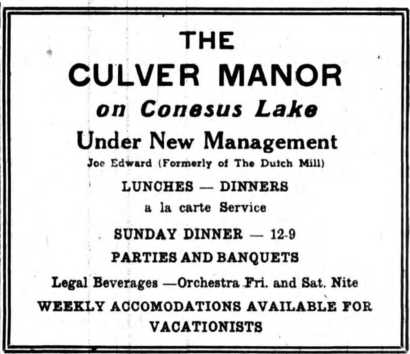This is a photo of a white sign with black text, bordered by a thin black and white double-line frame, taken outside a building. At the top center, it prominently reads "The Culver Manor on Knesset Lake" in bold font. Below this, in sequential order, the text announces "Under New Management" followed by "Joe Edward, formerly of the Dutch Mill." The sign details services such as "Lunches and Dinners, a la Carte Service," "Sunday Dinner, 12-9," "Parties and Banquets," and "Legal Beverages." Additionally, it mentions "Orchestra, Friday and Saturday night" and "Weekly Accommodations available for vacationists."